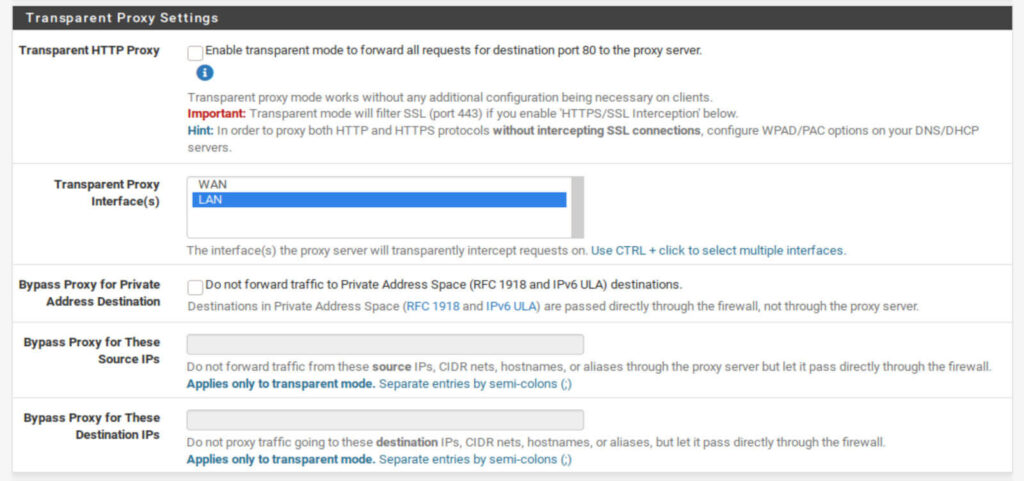This image displays the settings interface for Transparent Proxy Configuration. At the top, there is a grayish-black header labeled "Transparent Proxy Settings." Below it are five configurable sections:

1. **Transparent HTTP Proxy** - This section includes a checkbox to enable transparent mode, which forwards all requests destined for port 80 to the proxy server.
2. **Transparent Proxy Interfaces** - Here, you can select the interface through which the transparent proxy will operate, either WAN or LAN.
3. **Bypass Proxy for Private Address Destination** - This section features a checkbox labeled "Do Not Forward Traffic to Private Address Space (RFC-1918) and IPv6 ULA destinations." Enabling this option allows traffic destined for private address spaces to bypass the proxy server and pass directly through the firewall.
4. **Bypass Proxy for these Source IPs** - This area allows you to specify a list of source IP addresses that should bypass the proxy server.
5. **Bypass Proxy for these Destination IPs** - Similarly, this section lets you list destination IP addresses that will bypass the proxy server.

The detailed descriptions next to each option guide users in customizing how the proxy handles different types of traffic and addresses.